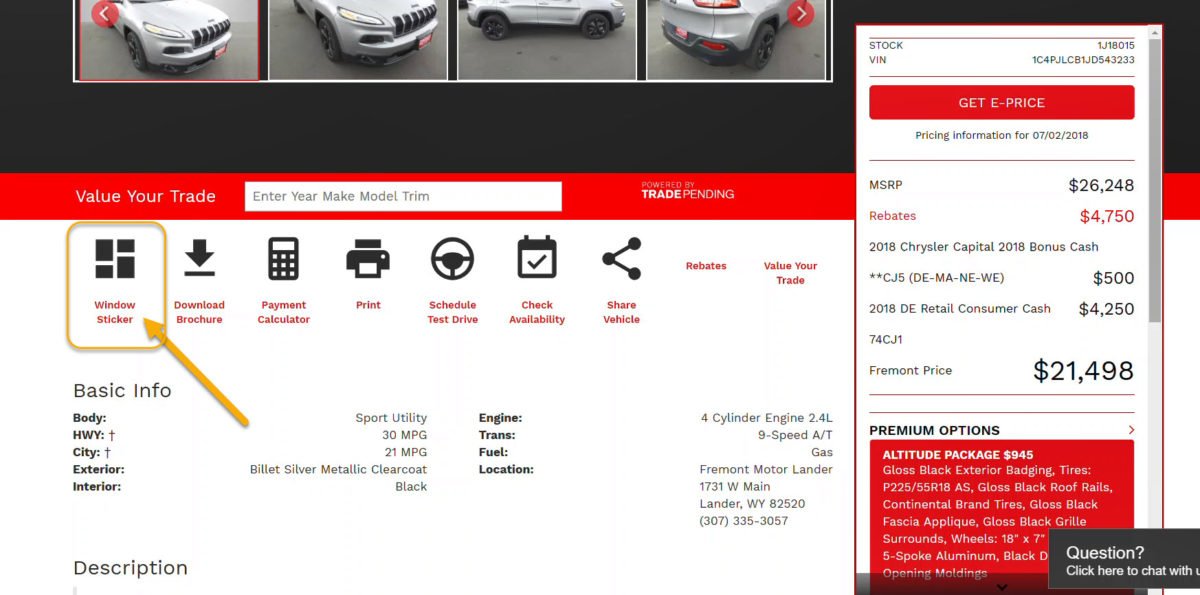A screenshot from a car dealership website, featuring a detailed display of a 2018 Chrysler Capital. The car is showcased through multiple images taken from various angles. Key information is prominently displayed:

- **Make and Model**: 2018 Chrysler Capital
- **Pricing**: MSRP is listed at $26,248, with a dealership price of $21,498.
- **Mileage**: 30 mpg (highway) and 21 mpg (city).
- **Exterior Color**: Billet Silver Metallic Clear Coat
- **Interior Color**: Black
- **Engine**: 4-cylinder engine

Additional features and options presented at the bottom of the screenshot include:

- **Window Sticker**
- **Download Brochure**
- **Payment Calculator**
- **Print**
- **Schedule Test Drive**
- **Check Availability**
- **Share Vehicle**
- **Rebates**
- **Value Your Trade**

Highlighted with an arrow is the "Window Sticker" option, drawing special attention to this feature for some reason.